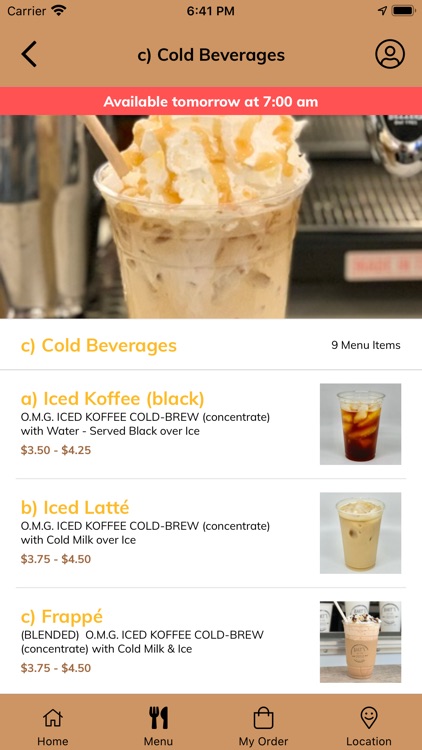The image depicts a web page displayed on a cell phone screen. At the top of the screen, the carrier information along with the Wi-Fi symbol and the time, 6:41 PM, are visible. There's an icon representing account access where users would sign in, indicated by a clickable circle. The title "Cold Beverages" is shown in a goldish-brown color with a less-than sign (<) to its left, suggesting a navigation option to go back.

Beneath this title is a coral-colored bar displaying "Available tomorrow at 7 AM" in white text. Below the bar, there is a high-quality image of a cold beverage, characterized by its whitish base topped with cream and drizzled caramel. The text "Cold Beverages" appears again in gold under the image, with a smaller print on its right stating "9 menu items."

The following section is a white area presenting three different beverages with their names and corresponding descriptions:

A. Iced Coffee
B. Iced Latte
C. Frappe

Each beverage listing includes a small thumbnail photograph and provides details such as the product description, price range, and minimum to maximum price. At the bottom of the screen, there is a gold navigation bar with options labeled "Home," "Menu," "My Order," and "Location."